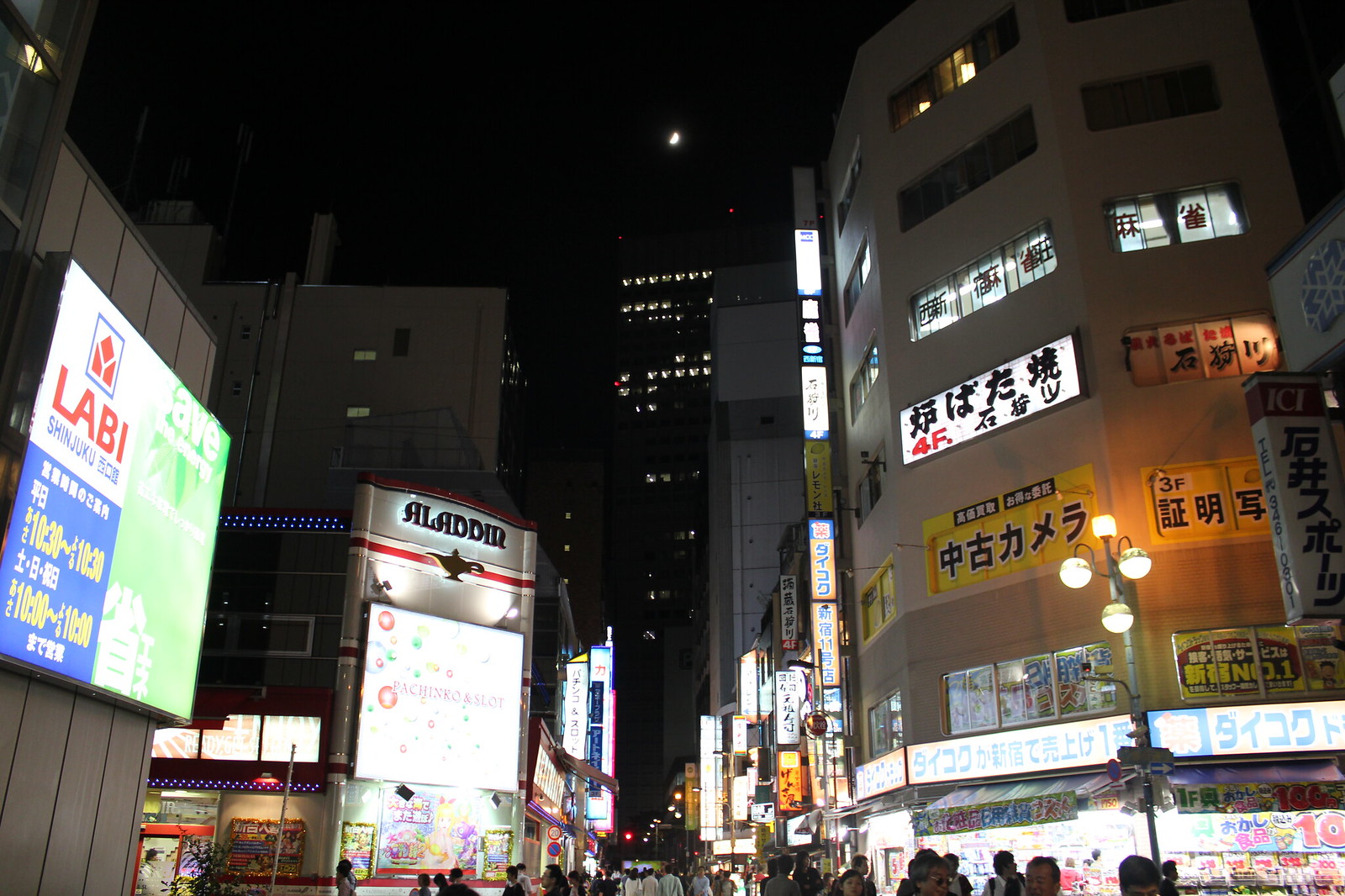The nighttime image captures a bustling downtown city street, framed by towering skyscrapers in the distance under a black sky. On either side of the street, mid-rise buildings stand, illuminated by various lights and signs. The left side of the street features a four-story building with a marquee reading "ALADDIR" and bustling activity at its base, where people are gathered and moving. Across the street on the right, a light gray building rises six or seven stories high, adorned with Asian characters on yellow banners covering some windows on the third floor, and an electronic board with more Asian characters on the fourth floor. Further right, a concrete building also displays Asian banners, adding to the eclectic urban scene. Digital displays showcasing different companies light up the street, reflecting in the windows of nearby storefronts. Close to the foreground, a large billboard marked with "L-A-B-I" in red letters and additional, indistinct characters draws the eye. The scene captures the vibrant, multifaceted essence of the city, with people mingling and exploring their urban surroundings.